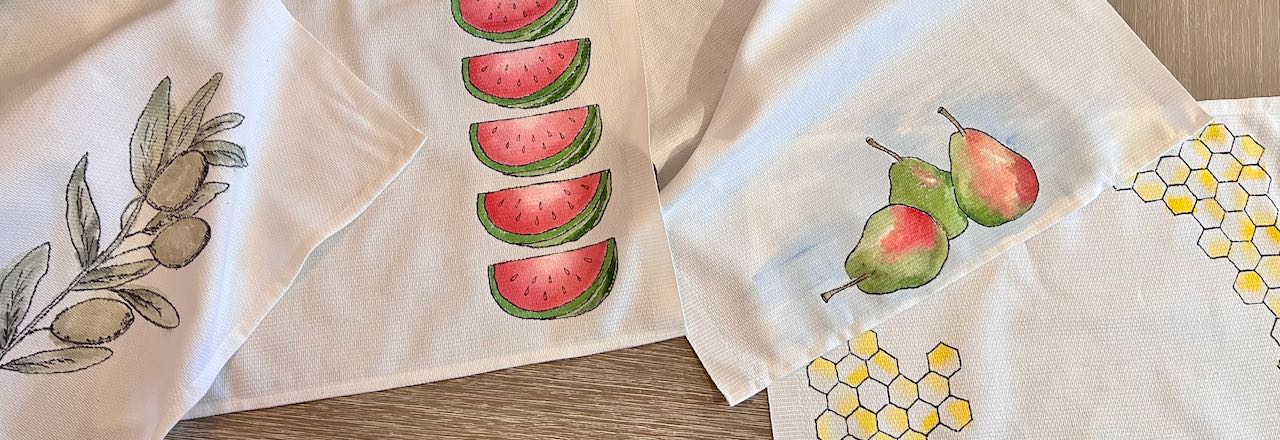This is an up-close photo of four cloth napkins laid out on a light wooden surface, each with distinct printed designs on a white background. 

On the left-hand side, a napkin showcases a sage-like or olive branch design, featuring three olives attached to a stem with leaves. To its right, the second napkin displays five neatly arranged watermelon wedges, all in a row. The third napkin in the sequence features three pears, shaded in green and red-orange; one pear is on its side while the other two stand upright. The final napkin in the lower right-hand corner has a design of yellow honeycombs decorating its borders.

The artwork on the napkins appears to be either hand-drawn or printed, contributing vibrant, natural-themed patterns to the ensemble.